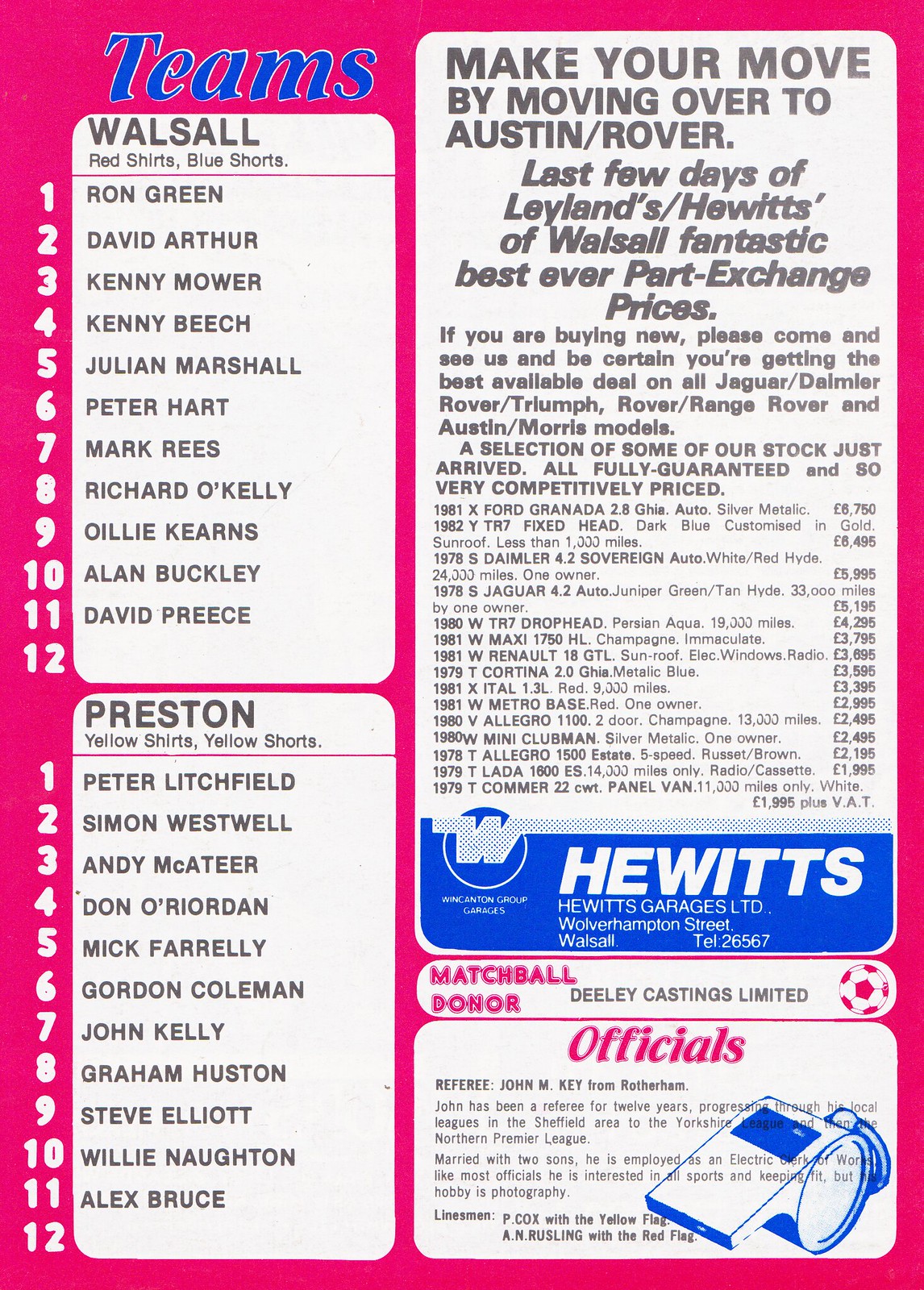The image appears to be a page from a game day program for a soccer match, set against a striking magenta to bright neon pink background. On the left side, there are two off-light to cream-colored text bubbles with rounded smooth edges, stacked vertically. Each bubble contains team information and player lists, enumerated from 1 to 12 in white script.

The top bubble lists the team Walsall, written in bold blue text with a white outline, followed by the text "red shirts, blue shorts" in gray script. The players listed include Ron Green, David Arthur, Kenny Moore, Kenny Beach, Julian Marshall, Peter Hart, Mark Rees, Richard O'Kelley, Ollie Kearns, Alan Buckley, and David Priest. Below Walsall, the second bubble details Preston, with "yellow shirts, yellow shorts" noted in gray script, and includes players Peter Litchfield, Simon West, Andy McKeeter, Don O'Riordan, Mick Farrelly, Gordon Coleman, John Kelly, Graham Huston, Steve Elliott, Willie Naughton, and Alex Bruce.

On the right side of the image is an advertisement within another off-light cream-colored bubble, featuring gray text: "Make your move by moving over to Austin Rover. Last few days of Leyland Hewitt's of Walsall's fantastic best ever part exchange prices." A detailed list follows, specifying various car models and their prices in euros, focusing on Jaguar, Daimler, Rover, Rover/Range Rover, and Austin Morris models.

Below the advertisement, another section mentions "Hewitt's Garage LTD" in white script against a medium to royal blue background, accompanied by a football logo in the far right corner labeled "Matchball donor, D-Link Hastings Limited."

At the bottom of the image, another white box with a blue whistle and the word "officials" rendered in pink, italicized text with a decorative sparkle effect, lists the referee John M. Key from Rotherham, along with other details.